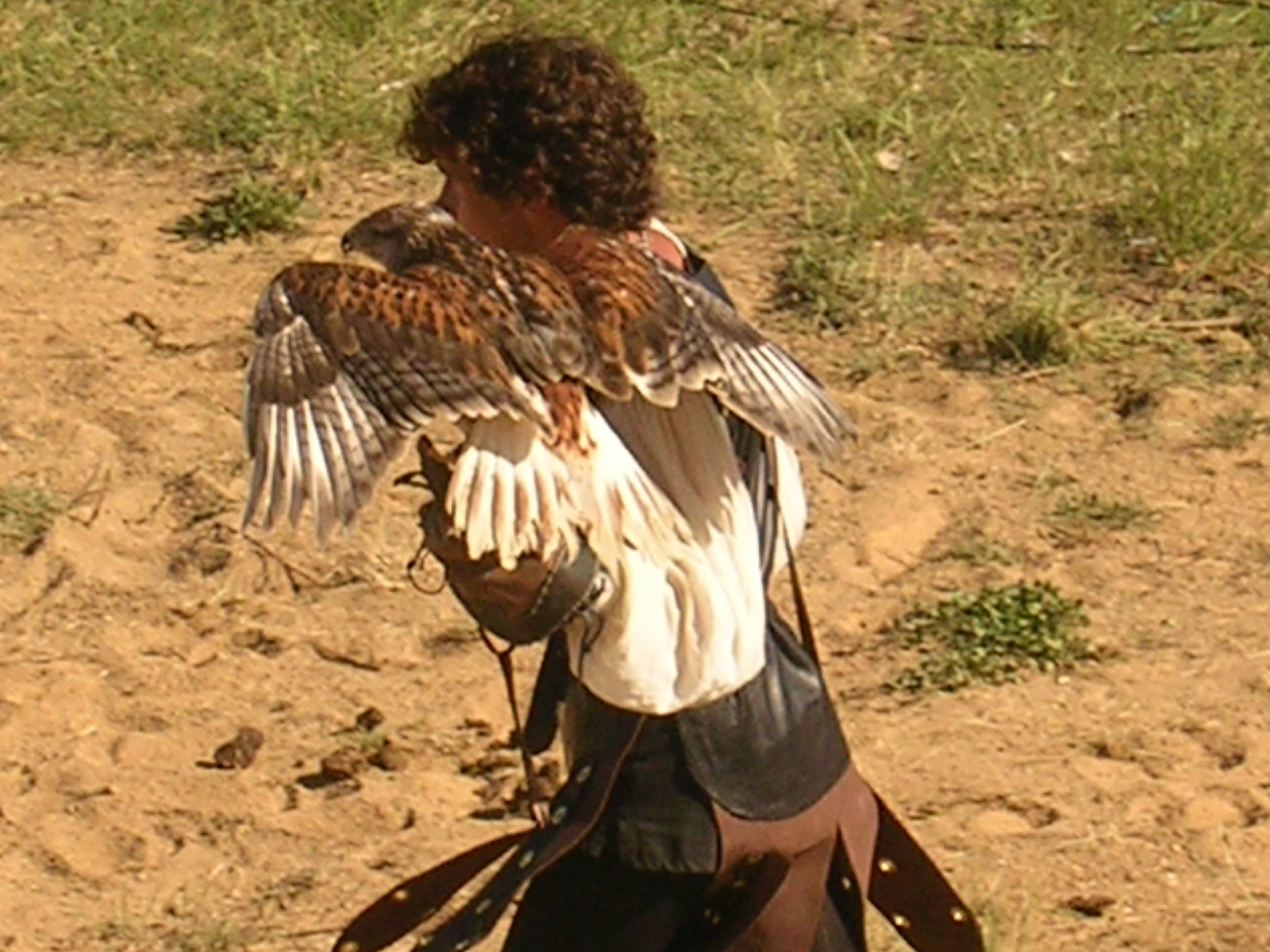The photograph captures a young, light-complected falconer with curly brown hair, centered in an outdoor, dry, and brushy landscape, possibly resembling regions like Arizona or Nevada. The ground is predominantly brownish dirt with sparse patches of grass, and some greenery is visible off to the side. The young man, possibly around 10 years old, is dressed in traditional falconry attire, featuring a white fluffy shirt, black leggings with a black skirt-like overlay, and leather straps around his waist. He wears a thick brown leather glove on his left hand, on which a hawk—possibly a falcon, adorned in brown feathers with black splotches and white-tipped wings—perches with its wings spread out. The scene is accentuated by the blending colors of beige, bronze, golds, whites, and creams, all bathed in daylight, providing a vivid and dynamic portrayal of the falconer and his bird in their natural setting.